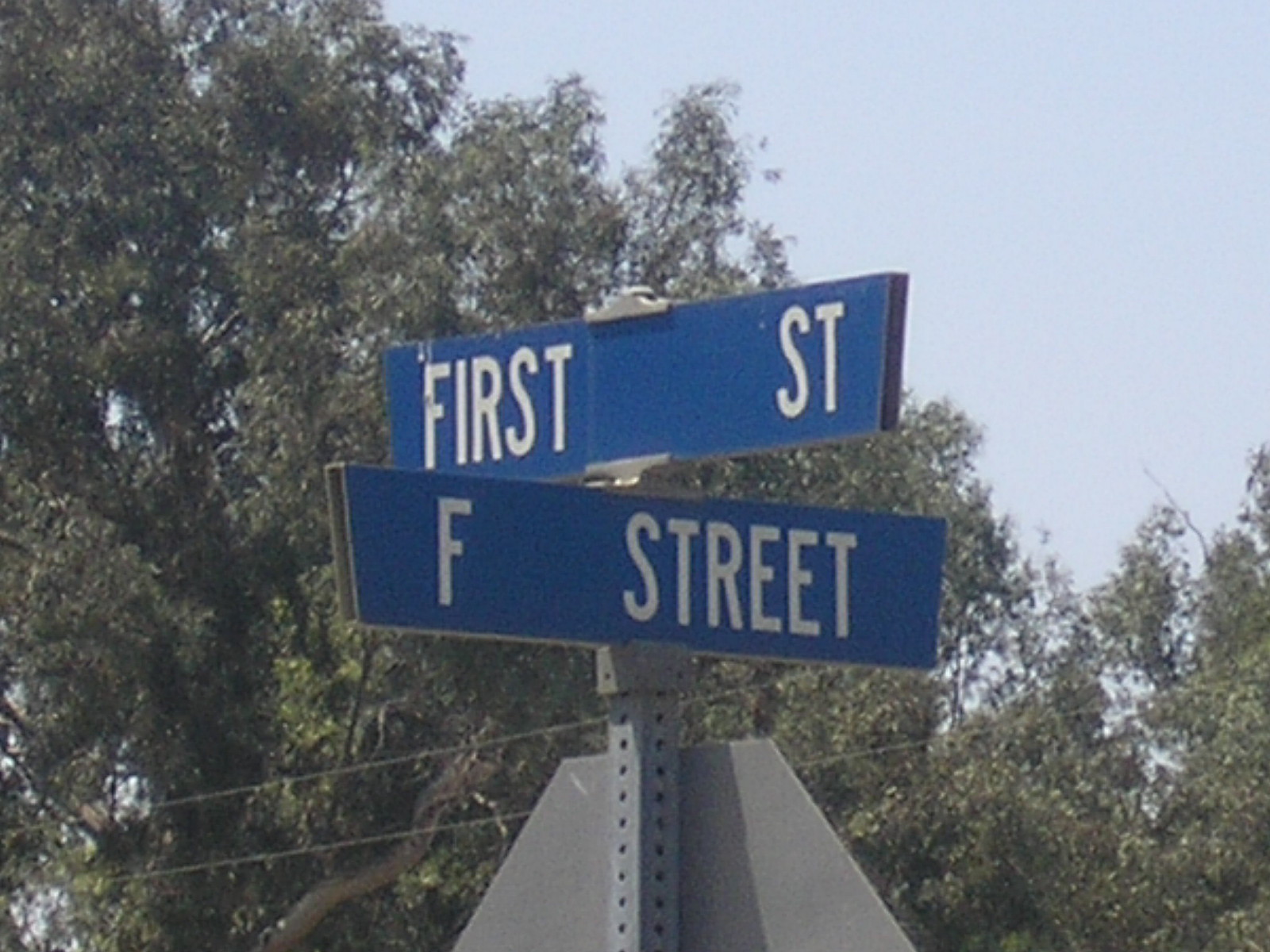This photograph captures an outdoor scene featuring two street signs mounted on a grey metal pole, which includes holes along its sides. The signs have a blue background with white, capital letters. The top sign reads "FIRST ST" and the bottom sign reads "F STREET." The "FIRST ST" sign appears to be missing some letters, suggesting they might have been removed or are in the process of being replaced. The scene is slightly grainy and blurred, indicating it might have been taken with an inexpensive device. In the background, a number of trees reach up towards a sky that varies in description, appearing grey in some accounts but noted as blue in others. Additionally, power lines or telephone wires are visible running through the trees. The image suggests a slightly vintage quality due to its overall graininess and slight blur.